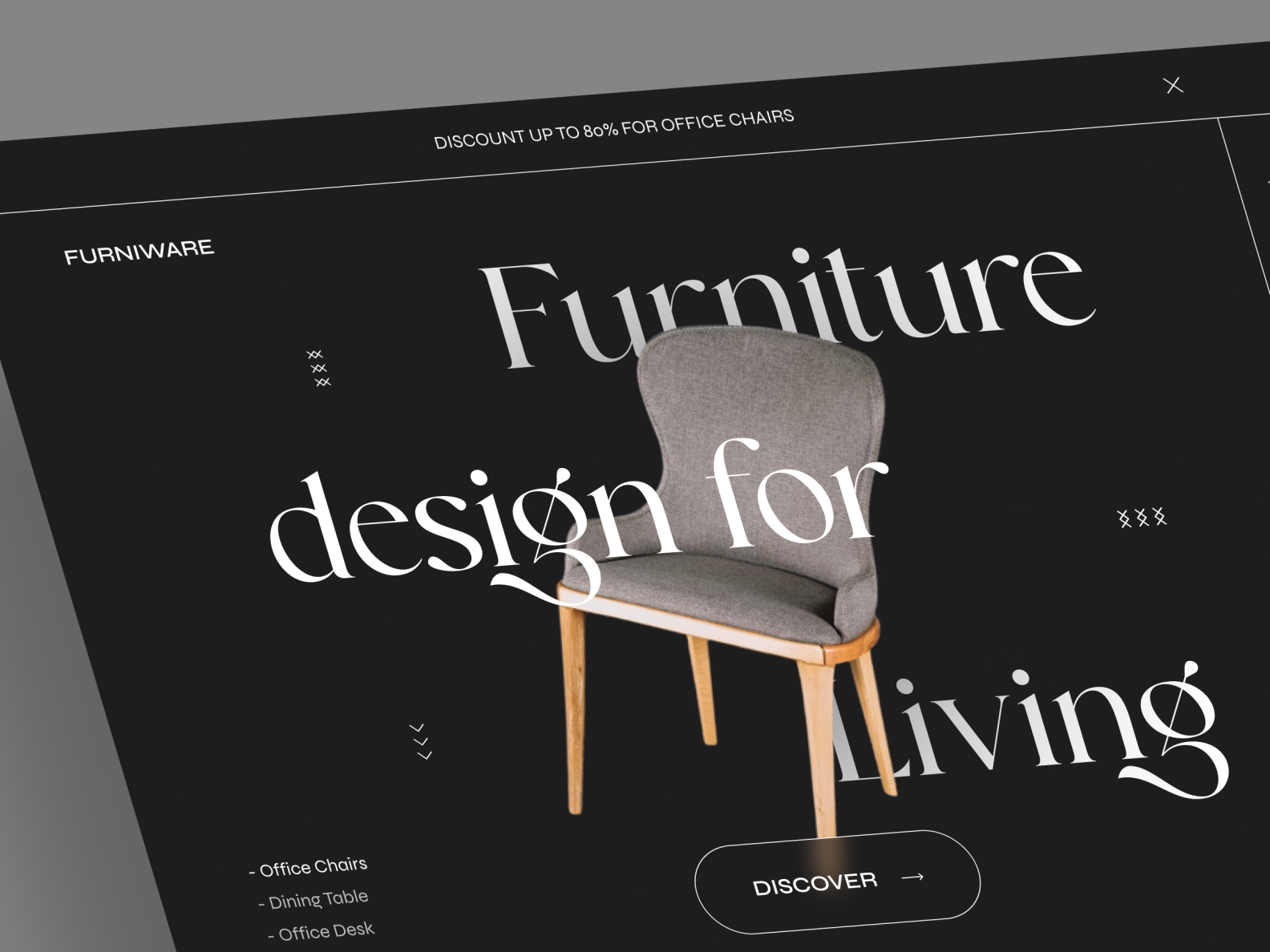The image captures a web page layout for a furniture retailer. At the very top of the page, there's a gray border that extends horizontally and vertically along the left side. The header section features a black background, prominently displaying a discount offer of "Up to 80% off office chairs" in bold lettering. Towards the far right of this section, there is a white "X" button for closing the pop-up, underlined by a solid white line.

The central portion of the image showcases an inviting photograph of a contemporary desk chair. The chair has a gray upholstered back and seat, with light wood legs offering a stylish and modern touch. Overlaying the chair image, the phrase "Furniture Designed for Living" is written in white text.

In the upper left corner, the brand name "Furnawear" is also displayed in white font. Directly beneath the chair image, an oval-shaped button labeled "Discover" along with a right arrow invites user interaction.

In the bottom left corner of the image, a navigation menu offers various categories: office chairs, dining tables, and office desks. The "office chairs" option appears to be highlighted, indicating the current view is focused on this category.